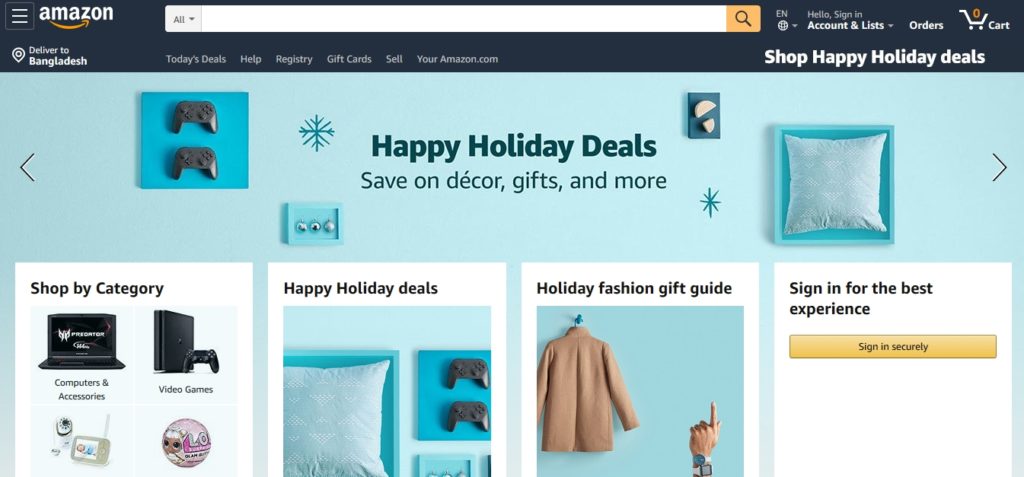**Detailed Descriptive Caption of the Amazon Page Screenshot:**

This screenshot captures the Amazon homepage with its characteristic dark blue theme, prominently visible at the top navigation bar. On the left side, the Amazon logo is displayed, featuring the word "Amazon" in black text with an iconic gold arrow forming a smile beneath it. Adjacent to the logo, there's a hamburger menu icon. Centered in the top navigation bar is the search box; a drop-down arrow beside the "All" text on the left and an orange block with a magnifying glass icon on the right suggest its functionality. To the right of the search bar are several elements: "EN" atop a globe symbol indicating language options, followed by "Hello, Sign in" above "Accounts & Lists" with a drop-down arrow, an "Orders" link, and a shopping cart icon showing "0" in gold, indicating no current items.

Right below the search bar, a location pin icon reads "Deliver to Bangladesh." The navigation text underneath includes links to "Today's Deals," "Help," "Registry," "Gift Cards," "Sell," and "Your Amazon.com." 

A promotional banner encouraging users to "Shop Happy Holiday Deals" in bold white text stands out on the right. The light blue background backdrop contains navigation arrows, a dark blue square with two black game controllers to the left, and a dark blue snowflake on the right, under which appears a light blue jewelry box lid with three silver balls inside. The center of the banner features a message in bold dark blue text: "Happy Holiday Deals," with a subtext in regular dark blue: "Save on decor, gifts, and more."

Further to the right, above the highlighted deals, a dark blue box with a strap contains an unidentifiable pink item resembling an ear. Below this is a smaller dark blue star or snowflake. To the far right is a lighter blue square depicting a light blue pillow.  

Below the banner are four predominantly white boxes showcasing various categories:

1. **Shop by Category**: At the top, black text reads "Shop by Category." Within a very light blue background, sections display "Computers & Accessories" alongside images depicting a laptop, a game console and controller (labelled "Video Games"), a security camera above a baby monitor, and a pink ball with a girl and musical notes inscribed with “LC.”

2. **Happy Holiday Deals**: Black text reads "Happy Holiday Deals" over a medium blue wall background. Featured items include a dark blue square with a light blue pillow to the right, another dark blue square with two game controllers to the left, and a light blue jewelry box top containing three silver balls (half cut off).

3. **Holiday Fashion Gift Guide**: This box in black text reads "Holiday Fashion Gift Guide." Against a medium blue background, a tan coat or jacket hangs from a blue thumbtack. Below is an image of a hand, with the sleeve strapped by a blue square and a black conversation balloon outline, showing the index finger pointing up.

4. **Sign In for Best Experience**: The last section displays a message in black text, "Sign in for the best experience," and a yellow "Sign in securely" button.

These elements create a detailed snapshot of the holiday-themed Amazon page, emulating the website’s comprehensive and user-friendly interface.